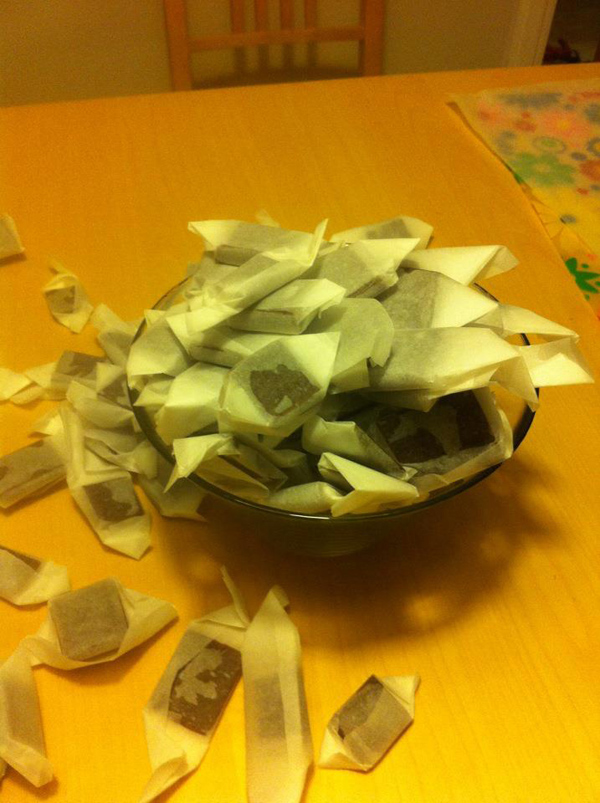This is a photograph of a dining room setup featuring a bowl of candies on a blonde pine wood table. The table has an oval shape with a visible armless pine dining room chair in the background, which has a cushion. To the right of the bowl, there is a piece of paper with a floral design displaying colors such as pink, green, and yellow. At the center of the image stands a glass or potentially clear or black bowl, overflowing with wax-wrapped candies. These candies are dark brown and black, rectangular in shape, and appear slightly greasy, giving a moist look through the wrappers. Some candies have spilled out of the bowl and lie directly on the tabletop, with their white wrappers partially unwrapped. The shot is taken from a perspective that captures the essential details of the dining setup, emphasizing the intricate floral design on the paper and the abundance of candies.